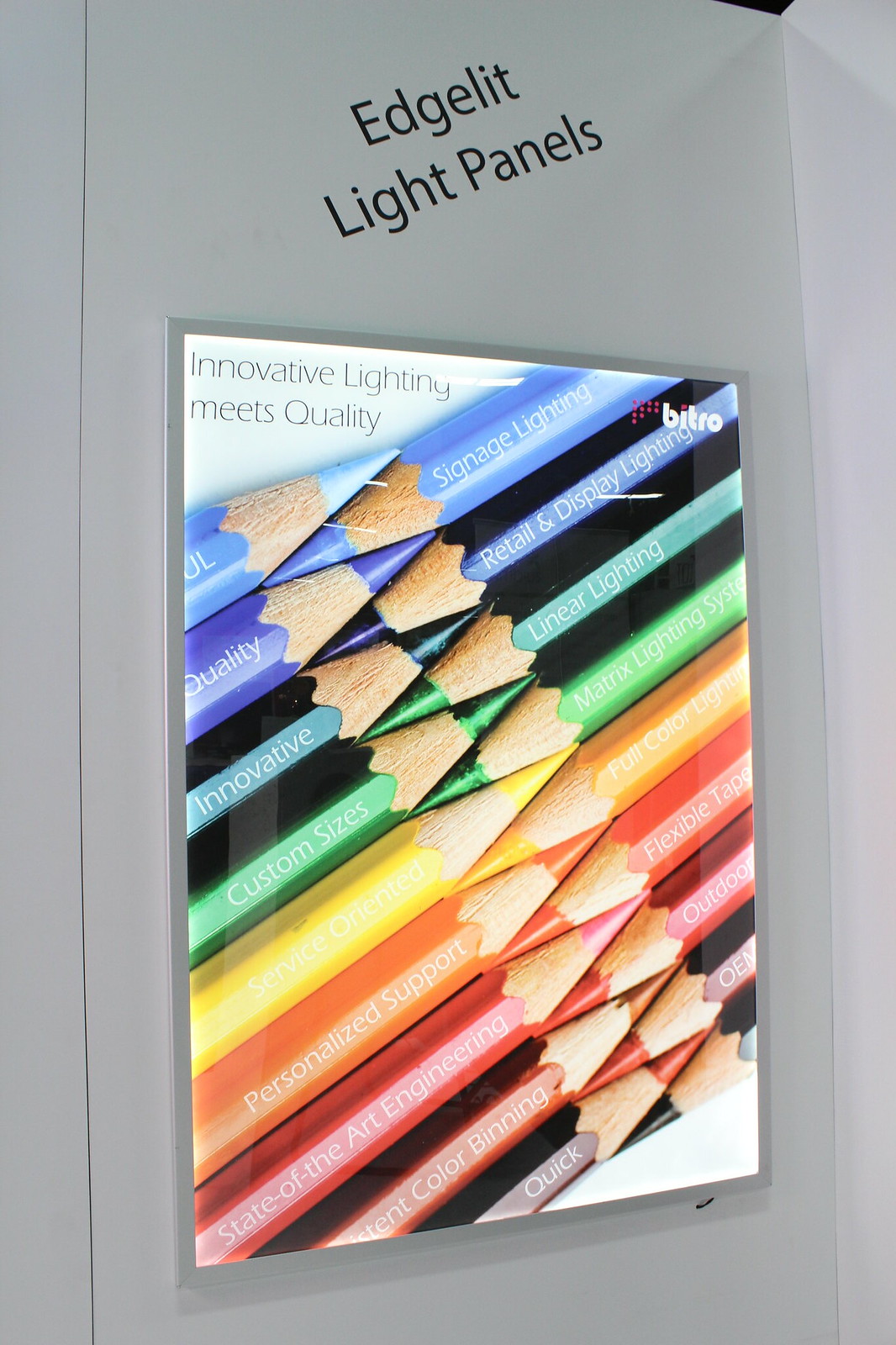This image showcases a detailed poster with a white background, displaying an array of interlocking colored pencils arranged diagonally from bottom left to top right. The pencils begin with dark red at the bottom, transitioning through shades of red, orange, yellow, green, blue, indigo, and ending with light blue at the top. Each pencil represents a different color in a gradient sequence, creating a rainbow effect. At the top left corner of the poster, the text "Innovative Lighting Meets Quality" is prominently displayed in black. Diagonally across the middle, in black type, are the words "Edge Lit Light Panels." Each pencil is labeled with terms related to lighting solutions, such as "Signage Lighting," "Retail and Display Lighting," "Linear Lighting," "Matrix Lighting," "Full Color Lighting," and more technical specifications. In the top right corner, the BITRO logo, consisting of the text "BITRO" and accompanying red dots, is positioned. The overall composition of the poster emphasizes a sophisticated integration of quality and innovative lighting technologies.